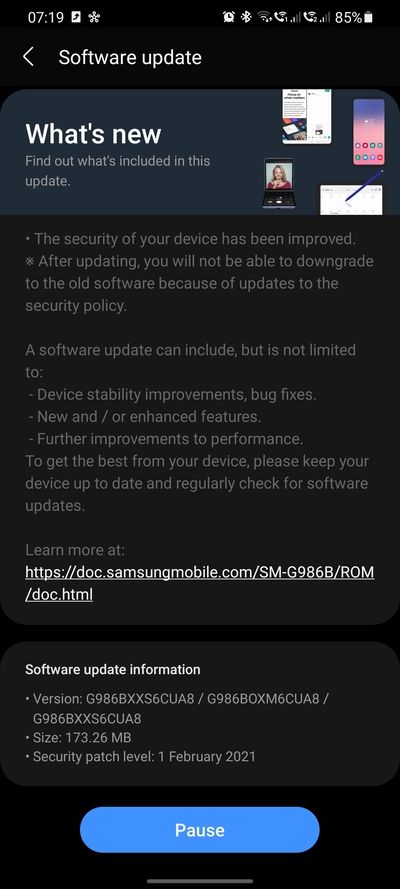The image depicts a cell phone screen displaying a software update notification. The background is entirely black, providing a stark contrast to the lighter colored text and icons, which are predominantly white, with some gray and light blue elements. In the upper left corner of the screen, the time, date, and a series of standard cell phone icons are visible, indicating the device's status and connectivity. Notably, the battery icon shows a charge level of 85%.

Below the header, the first option presented is "What's New," accompanied by four thumbnail images. These images give a preview of the updates included in the software package: one featuring a woman, another displaying a mockup of a cell phone screen with app icons, a third resembling a calendar with a pen poised to write, and a fourth not specified in the description.

Following the "What's New" section is a block of text regarding security updates. This section includes several lines describing enhancements and new features designed to improve the device's security. There's also a hyperlink labeled "Learn More," which directs users to a website offering detailed information about the security aspects of the update.

The notification concludes with details on the software update itself, including timing and additional pertinent information. The overall image is a comprehensive display of a typical software update notification on a cell phone, informing the user of the new features, security improvements, and update schedule.